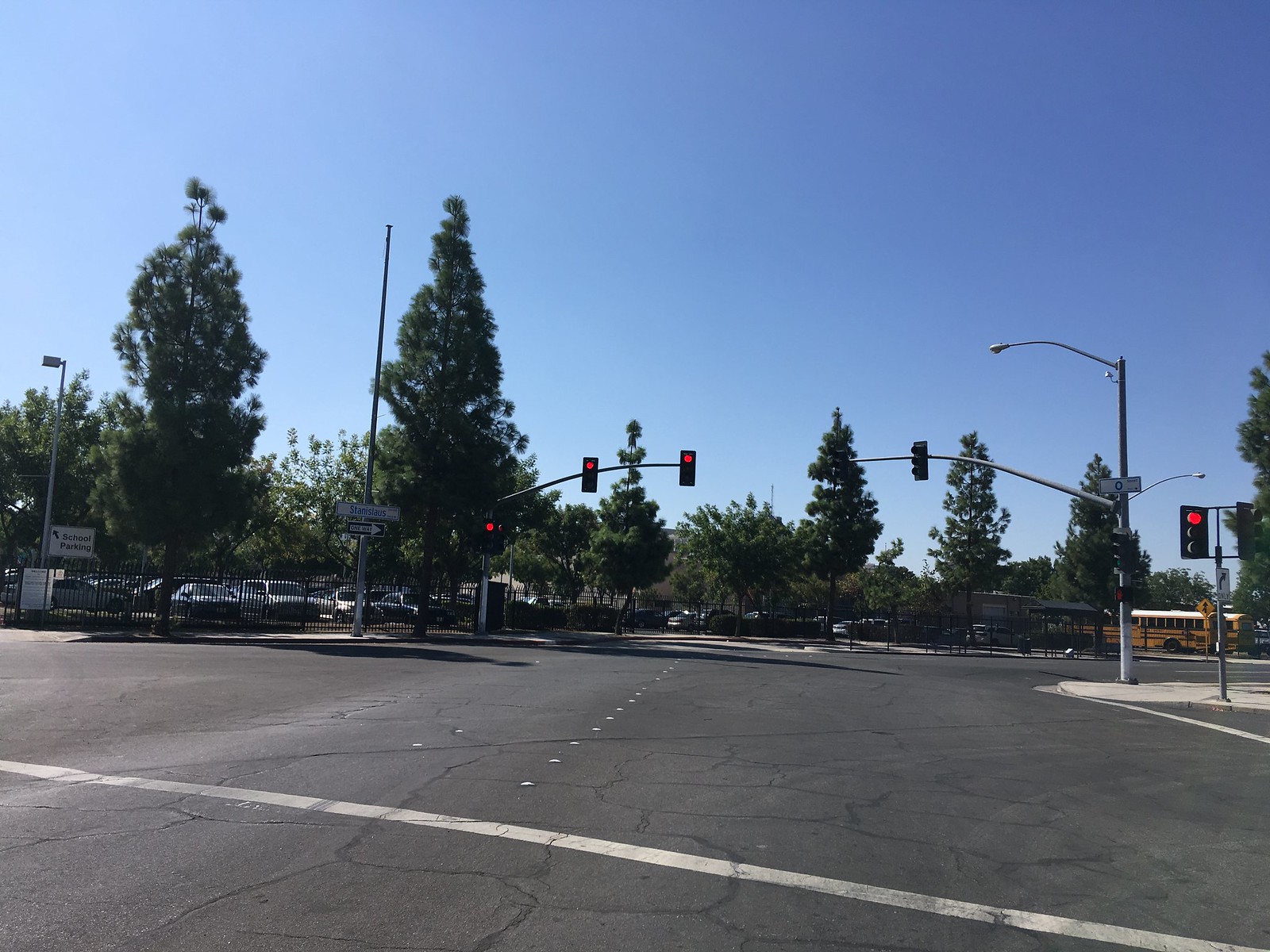In this vibrant urban scene captured during what appears to be spring or summer, the primary focus is a gray, weathered street marred by numerous cracks and dotted lines down the center. A prominent crosswalk line cuts horizontally across the street from left to right. To the mid-left of the frame, black railings are visible, potentially part of a pedestrian barrier. Adjacent to these railings sits a parking lot, filled with several parked cars. Along the far edge of the parking lot stand two line posts, one on the left and one in the middle.

Beyond the street and parking lot, the greenery of multiple trees is lush, suggesting the thriving vegetation typical of warmer seasons. The sky overhead is a strikingly bright blue, intensifying the overall daylight ambiance with sunlight emanating from the top left corner. This light casts a lively glow over the scene.

The street intersections are regulated by traffic lights positioned on both the left and right, with the latter extending midway across the road. All the visible traffic lights display red, signaling a complete halt. In the background on the middle right, a yellow bus with a white rooftop is partially visible, hinting at a school zone or public transport route. Directly below this bus, the sidewalk is seamlessly accessible with a curb cut, facilitating ease of pedestrian movement.

Further enhancing the scene are multiple lampposts, including one directly above the bus stop, which has a canopy and seating area for waiting passengers. The daylight renders the lamppost's light unnecessary. Additionally, subtle details like skid marks on the road indicate active vehicular use, adding to the dynamic nature of the urban landscape.